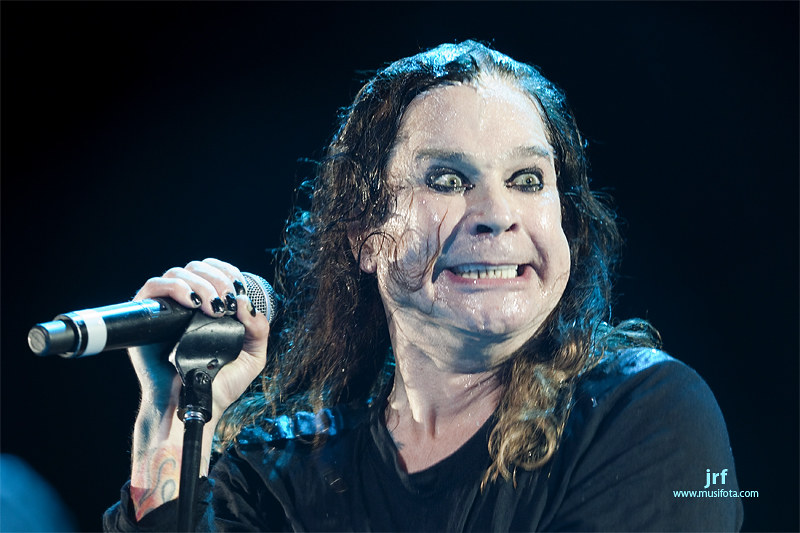This photograph features what appears to be Ozzy Osbourne caught mid-performance. The image centers on him from the chest up, against a completely black background. He grips a black microphone with a green detail in his left hand, which rests on a stand. His fingers are adorned with black nail polish. He's dressed in a simple black t-shirt, bringing attention to his characteristically long, thin, and greasy hair that cascades past his shoulders. His face is painted to appear unnaturally pale with heavy black eyeliner emphasizing his eyes, creating a dramatic and intense look. Osbourne's expression is a menacing grimace, and his eyes are wide and directed to the right, adding to his wild and eccentric appearance. His face glistens with sweat, enhancing the intensity of the moment captured. Near the bottom right corner of the image, in blue font, the text reads "JRF www.mucifota.com". Additionally, the shoulder of another person is faintly visible in the bottom left corner.